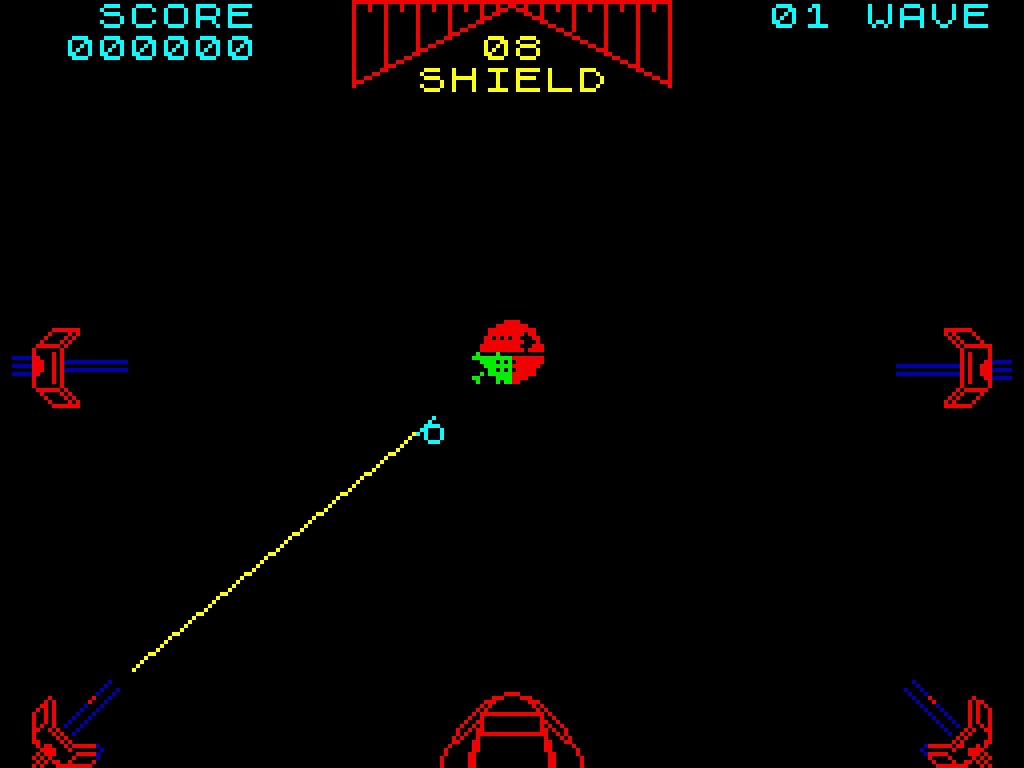The screenshot depicts a scene from a vintage arcade video game, seemingly a Star Wars title from the mid-1980s, potentially linked to "The Empire Strikes Back." The interface features a distinctive retro aesthetic with vector graphics. At the top center, a red rectangular box filled with intricate lines displays the text "08 SHIELD" in yellow below it. The top left corner shows the word "SCORE" followed by a series of six zeros indicating the current player score. On the top right, the display reads "01 WAVE," suggesting the current level or wave the player is on.

Centered on the screen is a prominent red circle, which might represent the Death Star, a key element from the Star Wars universe. Flanking this central icon, smaller red line drawings appear in the top right, top left, bottom left, and bottom right corners of the screen. Additionally, a larger red line drawing occupies the bottom center of the display. A bright yellow line extends diagonally from the bottom left feature to the central red circle, adding a dynamic visual element to the image. These graphical elements together create a compelling snapshot of the game's interface, evoking a strong sense of nostalgia for the arcade era.